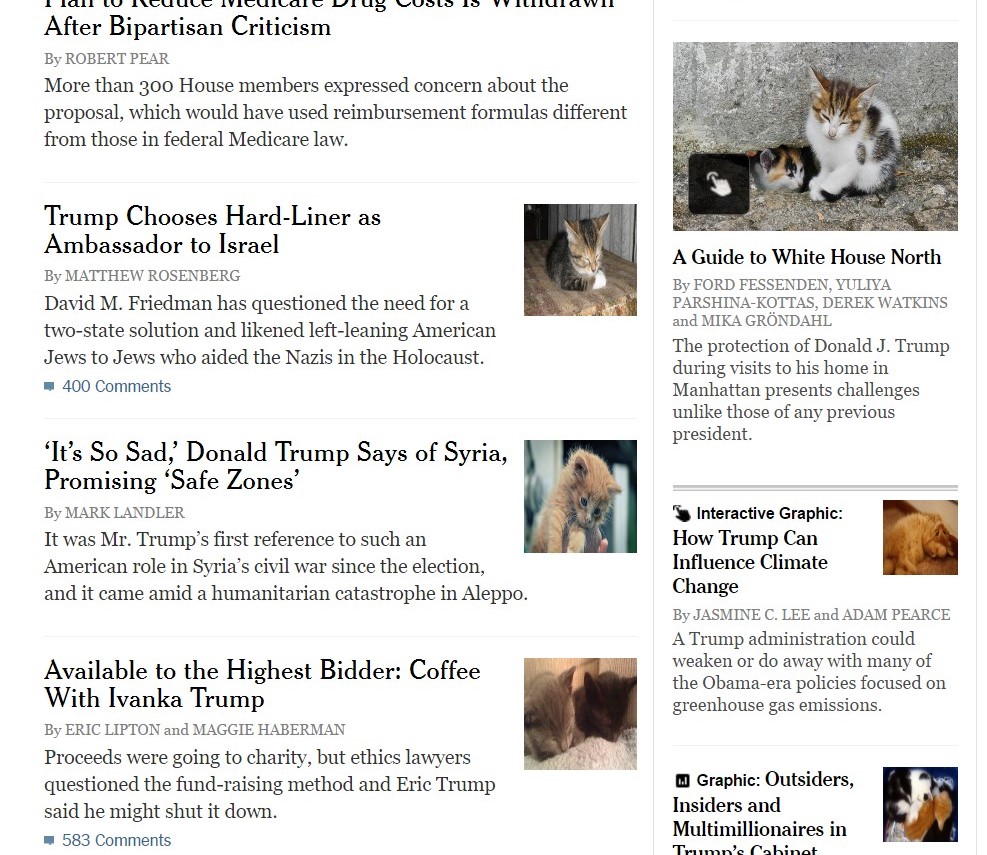The webpage in the image appears to be a news aggregation site, showcasing a variety of current articles. Notably, many of these articles include colorful photographs of cats and kittens, which do not seem to be directly related to the news stories. 

1. Trump Appoints Hardliner as Ambassador to Israel.
2. "It's So Sad," Trump Says of Syria, Promising Safe Zones.
3. Coffee with Ivanka Trump Available to the Highest Bidder.
4. An Interactive Graphic on How Mr. Trump Can Influence Climate Change.
5. A Guide to the White House's North: The Challenges of Protecting Donald Trump During Manhattan Visits.

Seven articles are visible in total, though the headline of one appears to be truncated. The articles seem reputable despite the incongruous kitten imagery. The kittens are prominently displayed in full-color photographs, adding a curious visual distraction from the serious topics discussed.

This descriptive caption should give a clear and detailed overview of the webpage’s content.